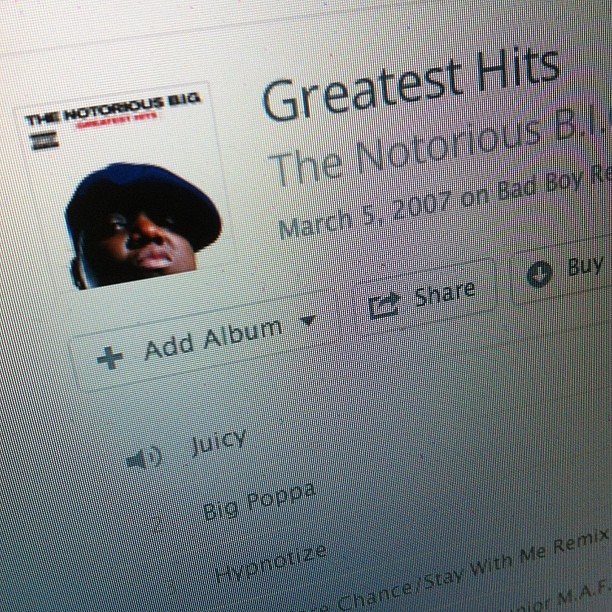The photograph depicts a rectangular computer screen, most likely a laptop, showing an album listing for "Greatest Hits" by The Notorious B.I.G., released on March 5th, 2007, under Bad Boy Records. The screen background is white. At the top of the screen, the album title "Greatest Hits – The Notorious B.I.G." is prominently displayed in black text. Beneath the title is the album cover, featuring an image of The Notorious B.I.G. wearing a black hat that casts a shadow over the left side of his face as he looks directly at the camera. Below the album cover and artist's name, there are three interactive buttons: "add album," "share," and "buy." Under these buttons, part of the tracklist is visible, listing the top three songs: "Juicy," "Big Papa," and "Hypnotize." The text and buttons on the screen are displayed in black and gray, maintaining a cohesive and clean visual layout.